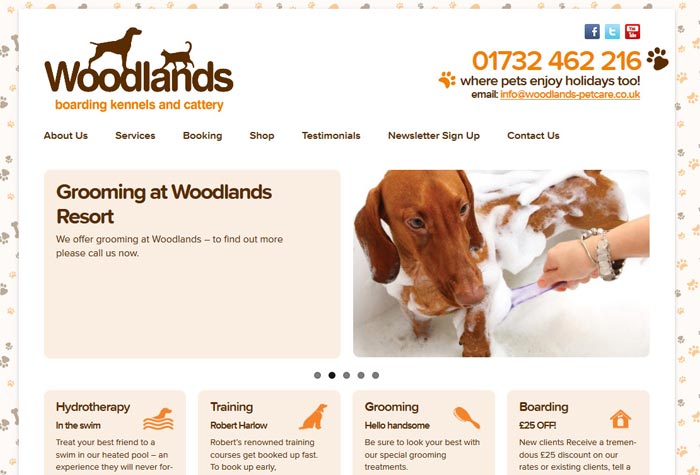The screenshot showcases the website for Woodlands Boarding Kennels and Cattery. In the top left corner, the brand name "Woodlands" is displayed in brown, accompanied by an icon of a dog and a cat. Beneath it, the text "Boarding Kennels and Cattery" is written in orange. On the top right, there are icons for Facebook, Twitter, and an unidentified red social media platform, next to the contact number 01732-462-216, which is adorned with brown and orange paw prints. The tagline "Where Pets Enjoy Holidays Too" is followed by the email address info@woodlands-petcare.co.uk.

The navigation menu includes links for About Us, Services, Booking, Shop, Testimonials, Newsletter Signup, and Contact Us. Below the menu, a section titled "Grooming at Woodlands Resort" invites visitors to call for more information about their grooming services. 

An image features a predominantly brown dog with white patches being bathed by a woman using a purple scrub brush, her wrist adorned with bracelets. The dog is covered in white bubbles, indicating a thorough clean.

Further down, four boxes outline the various services offered: Hydrotherapy with a drawing of a swimming dog, Training with a picture of a dog, Grooming with a brush icon, and Boarding with a house icon.